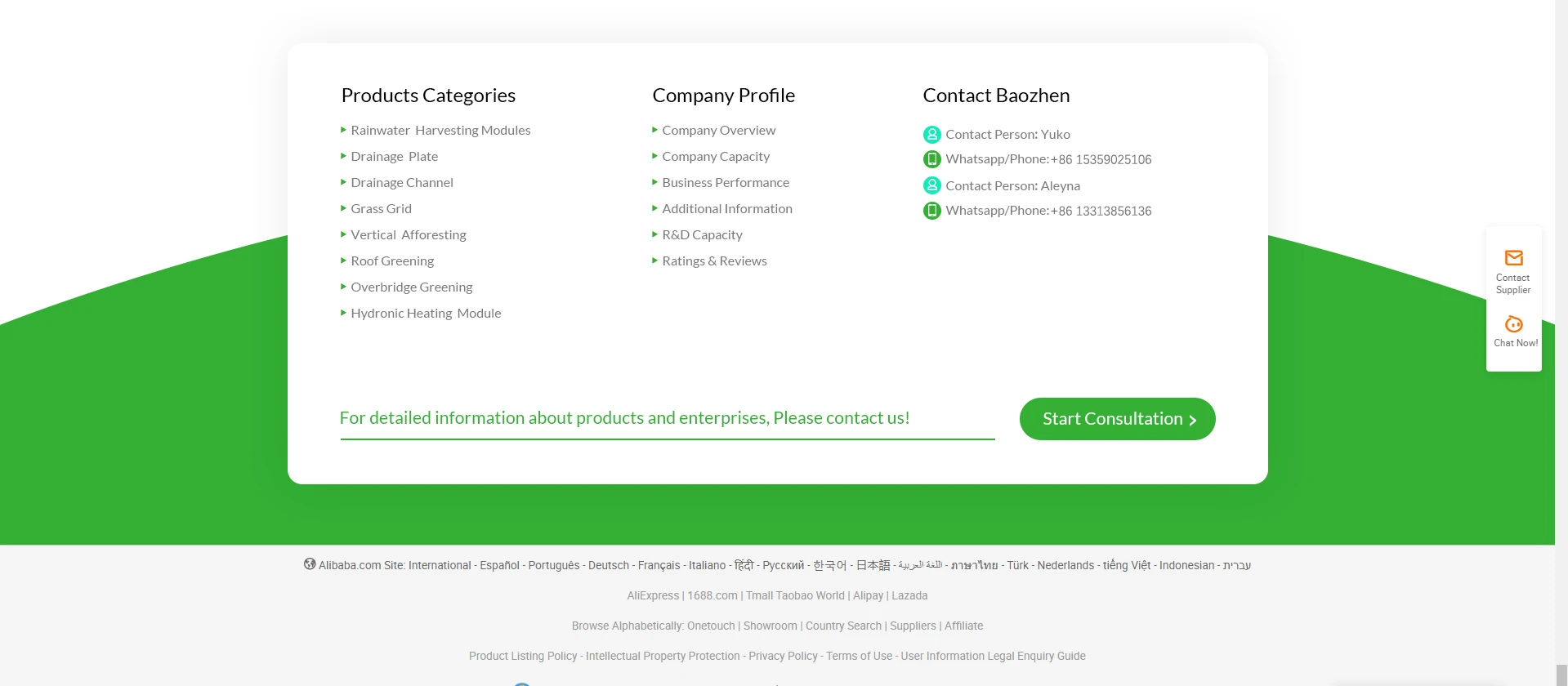The image depicts the bottom section of a generic business consultation website. The lower part of the webpage features various links and detailed product categories, such as "Rainwater Harvesting Modules" and "Drainage Channels," presented in small font. Additional sections include "Roofing," a "Company Profile," "Company Overview," and "Company Capacity." Contact details are prominently displayed, with multiple phone and WhatsApp numbers listed for inquiries. A notable call-to-action for more detailed product and enterprise information is highlighted with a large green button labeled "Start Consultations." Beside it, there are two more buttons on the right, which appear embedded but are not legible in the image. The design includes a simplistic white and green theme, with a gently curving convex green hill as part of the visual motif. Further down, the image contains more contact information and legal details, typically found in the footer section of a website.